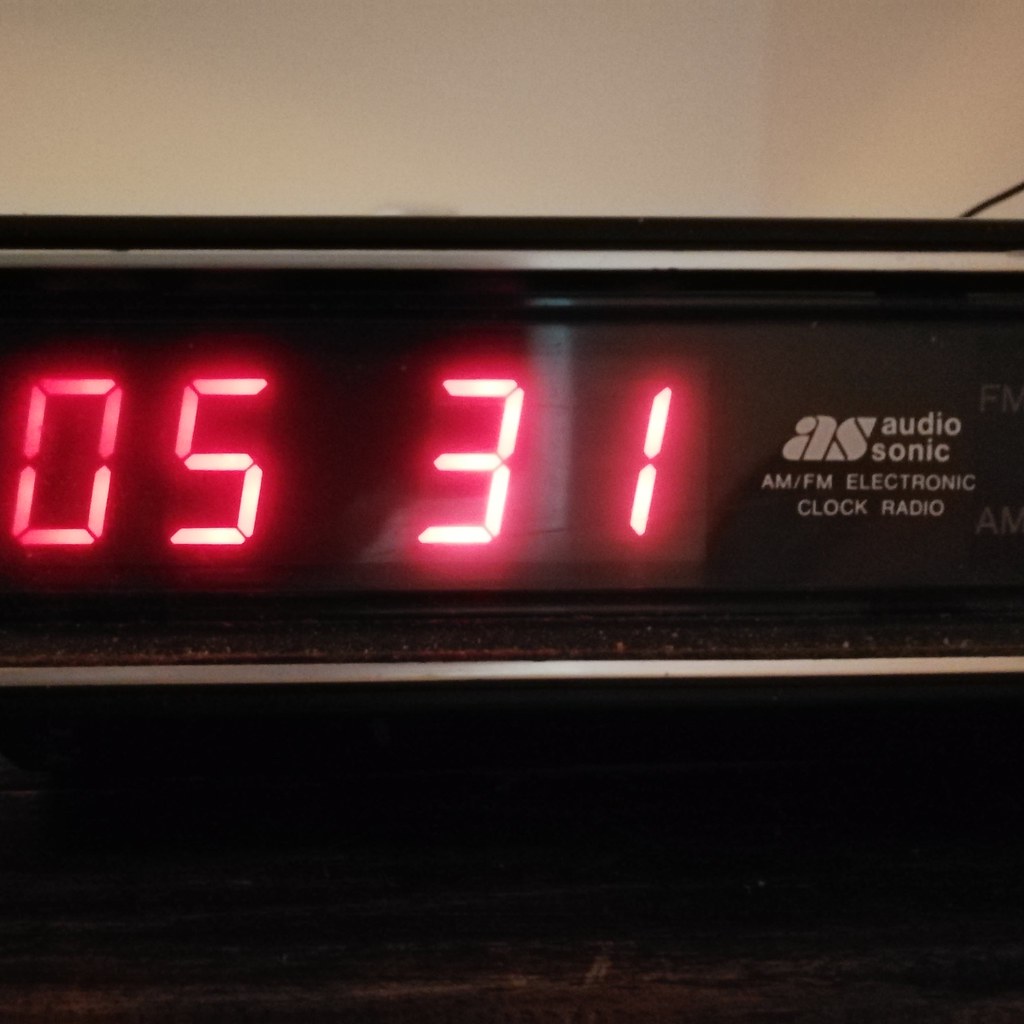The image is a close-up of a vintage digital clock radio, showcasing its sleek design. The digital display prominently features red LED numbers indicating the time as 5:31. The device is manufactured by Audio Sonic, a company known for its AM-FM electronic clock radios, likely from the 1980s or 1990s. The clock is positioned on a dark surface against a stark white wall, which contrasts sharply with its own darker casing and accentuates its retro aesthetic. The image captures the nostalgia and classic appeal of a bygone era in consumer electronics.